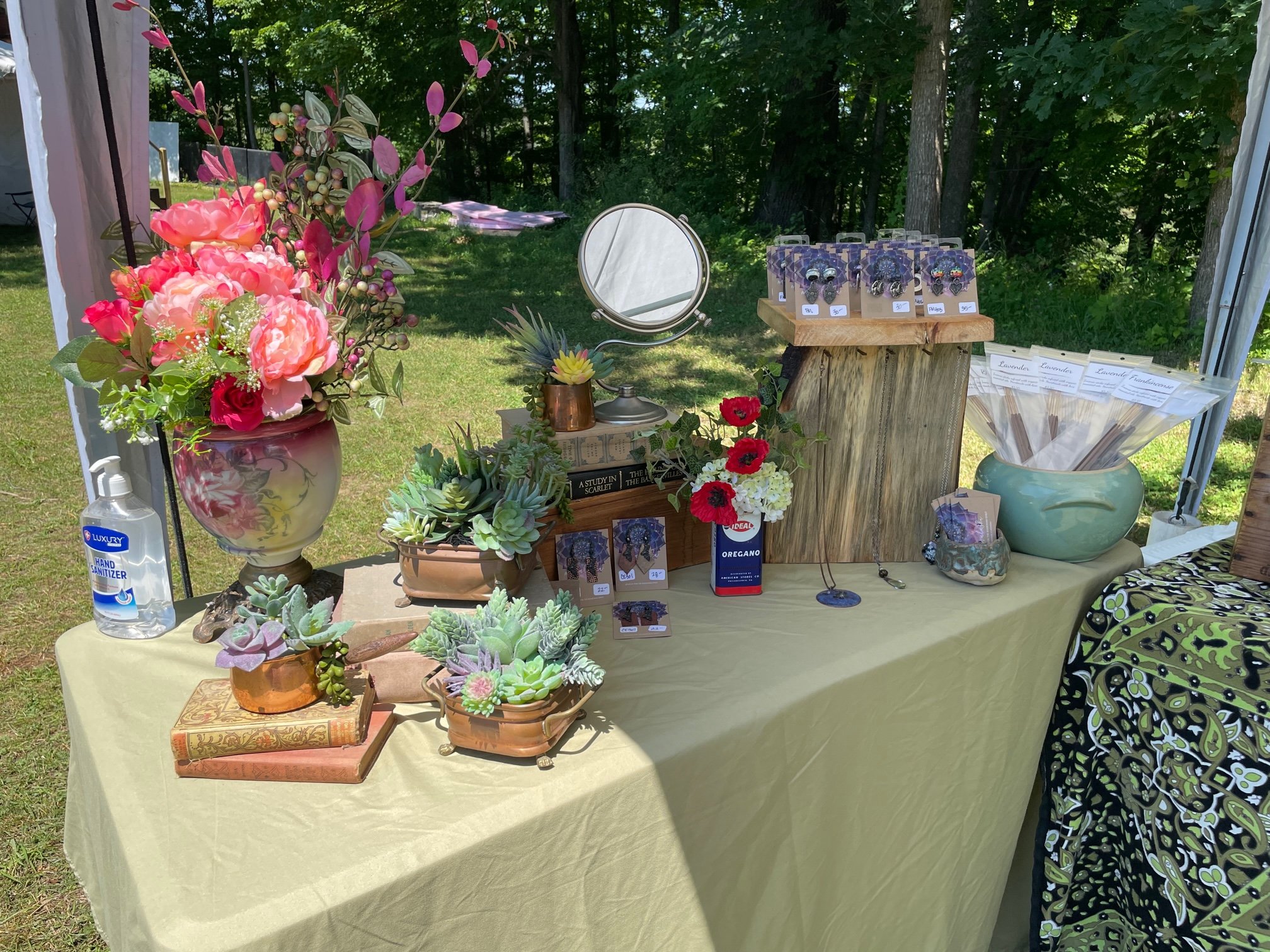The image shows a rectangular table covered with a beige or tan tablecloth, set up as part of a booth at an outdoor event, likely a farmer's market, boutique fair, yard sale, or outdoor festival. The table is situated under a canopy structure, with trees and grass visible in the background. 

On the table, a large bottle of hand sanitizer is placed on the far left. A vibrant and colorful vase overflowing with a beautiful arrangement of pink peonies and various green foliage adds a fresh, inviting touch. There are several pots of succulents positioned around the table, some placed on top of decorative books. Displayed on the table are earrings, alongside pricing labels presented in a blue vase-like bowl. Incense sticks are organized in a large green pot, with what appear to be incense cones or possibly more earrings placed nearby. A large mirror stands on top of some books, serving as a utility for customers to try on earrings. Overall, the table is artistically arranged with a blend of decor and items for sale, creating an inviting and aesthetically pleasing display.